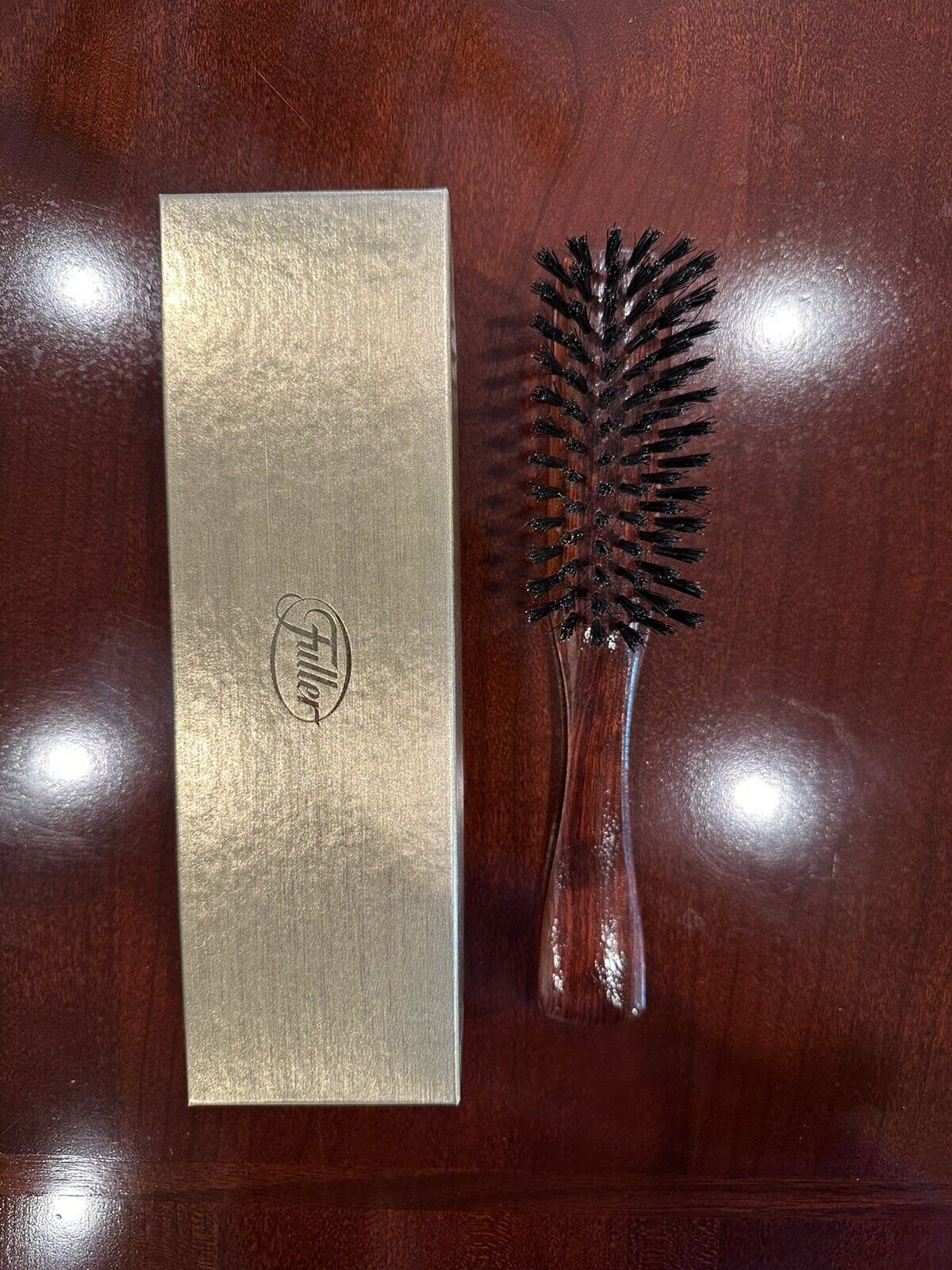The image depicts a shiny brown hairbrush with black bristles resting on a dark wooden platform. The platform, which has a reddish tint, features five white light spots reflecting off its surface. To the left of the brush lies a box, which is predominantly gold with silver hues. The box, which likely contained the brush, has the word "Fuller" engraved on it, set within an oval outline. Both items—the brush and its box—are arranged to emphasize the contrast between the dark wood and the reflective surfaces of the brush handle and the box.